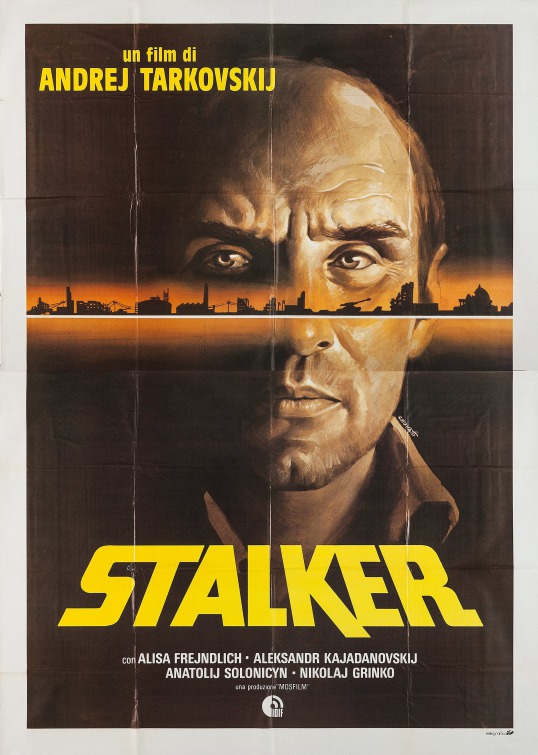This vertically aligned rectangular poster features a dark brown background with a striking central element: the face of an older, bald man with slightly shaggy brown hair on the sides, giving off a serious expression. His face is split horizontally by a white line, along which runs a narrow horizontal band with an orange glow, depicting a silhouette of military vehicles, tanks, factory buildings, and smokestacks. This industrial imagery intersects his eyes from above and his nose and mouth from below, where his face fades into the background. The upper left corner of the poster contains yellow text that reads "Un Film D'Andrzej Tarkowski," indicating it is a foreign film. Across the bottom center, in bold, angled yellow letters, the title "STALKER" is prominently displayed. The poster is worn, showing visible fold marks that divide it into a grid with eight squares down and four across.